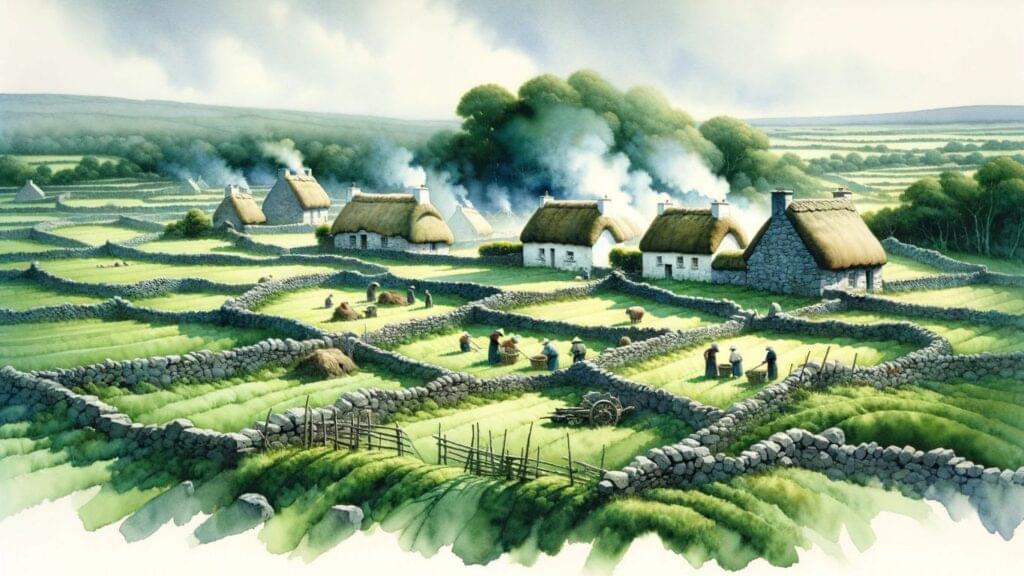This highly detailed watercolor painting vividly captures a tranquil English countryside farm. The predominant green hues highlight the vast stretches of rolling grass and hills, while the artist has delicately bled out the colors at the bottom of the canvas, adding a soft, unfinished touch. The farmland is meticulously sectioned with rock and stick fences, delineating various pastures and fields where farmers are diligently working with rakes, baskets, and other equipment. Some are seen creating haystacks and interacting with stacks of hay. Scattered farming tools and a wagon further enrich the rural atmosphere.

Whitewashed and cobblestone houses with straw roofs dot the top third of the painting. The quaint homes, some emitting smoke from their chimneys, add a lived-in charm to the scene. The sky, a wash of mostly white with hints of blue and discoloration from the smoke, looms quietly above. In the background, billowing smoke suggests a central fire or multiple chimney emissions near a cluster of trees and ridges. Beyond, the landscape unfolds into more green pastures and distant hills, encapsulating the serene essence of the English countryside.